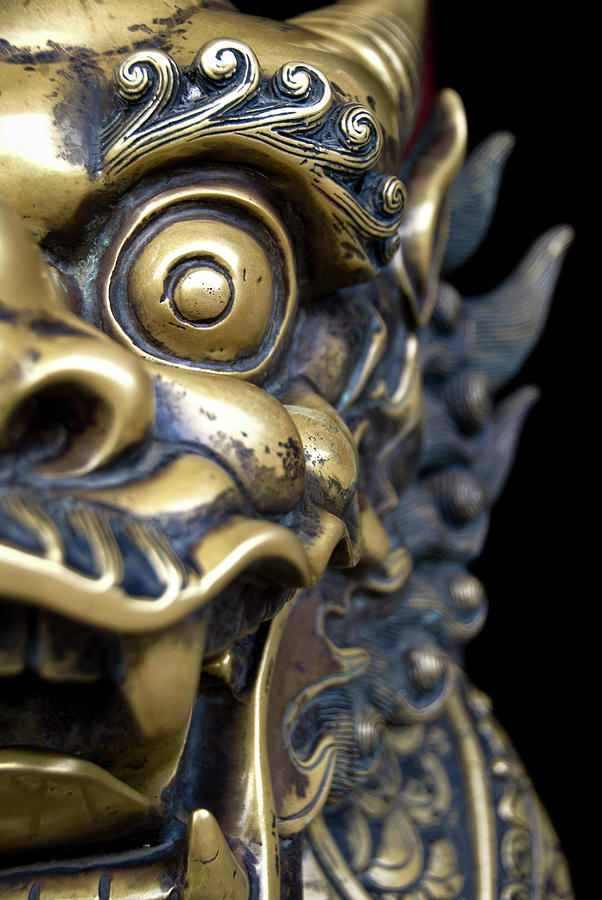This detailed close-up photograph showcases the left side of an aged Chinese dragon statue, set against a dark black background. The statue is crafted from a light brown metallic material with signs of patina—blackened creases indicating wear and oxidization, contrasting with its golden-bronze hues. The dragon's face is characterized by a broad nose with large, flared nostrils and very expressive, wave-like eyebrows made up of curled hairs. Its rounded eyes are strikingly colored in gold and blue, with the left eye prominently featured. The dragon's open mouth reveals humanoid teeth, including a distinct gold tooth. The statuesque creature also possesses a sharp, blue-tinted mane that accents its formidable appearance, further enhancing the intricate artistry and antique allure of the sculpture.